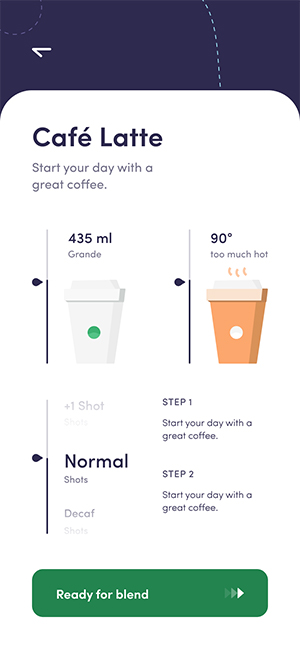This image features a digital interface of a coffee preparation app designed to customize your morning coffee experience, specifically focusing on a Café Latte. The interface provides three primary customization options. 

1. **Volume Selection**: Users can choose the amount of coffee in milliliters, allowing for precise control over their desired quantity.
   
2. **Temperature Control**: The app offers an adjustable temperature setting, initially set at 90 degrees Fahrenheit, with a note that the current setting is "too hot." Users can scale the temperature up or down to achieve their preferred warmth.

3. **Strength and Type Options**: There are selections for the coffee's strength and type, including "normal," "decaf," and an additional option for a "plus one shot." This allows users to specify their caffeine preference.

Notably, the interface also repeats the initial prompt, asking, "How would you like to start your day with a coffee?" and "Start your day with a great coffee," emphasizing the user’s choice.

At the bottom of the display, a prominent green button labeled "Ready for blend" is present, guiding users to finalize their customizations. Accompanied by white arrows indicating progression, clicking this button is expected to advance the user to the next step in the coffee-making process.